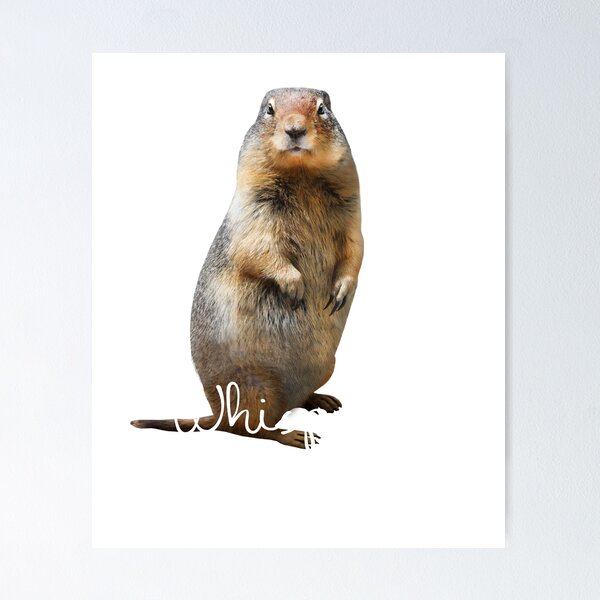The image depicts a beaver standing on its hind legs, facing and looking directly at the camera with an expression that almost seems to ask, "What do you want?" The background is entirely white, which makes the beaver the sole focus of the image. The beaver's fur is a mix of black, brown, and off-white, with a reddish-brown area covering its nose up to the eyes and extending to its chest. Its claws are long and visible, and its tail can be seen trailing behind. There's a white piece of paper with a faint script in white cursive at the bottom, reading "WHISP," difficult to discern against the white background.